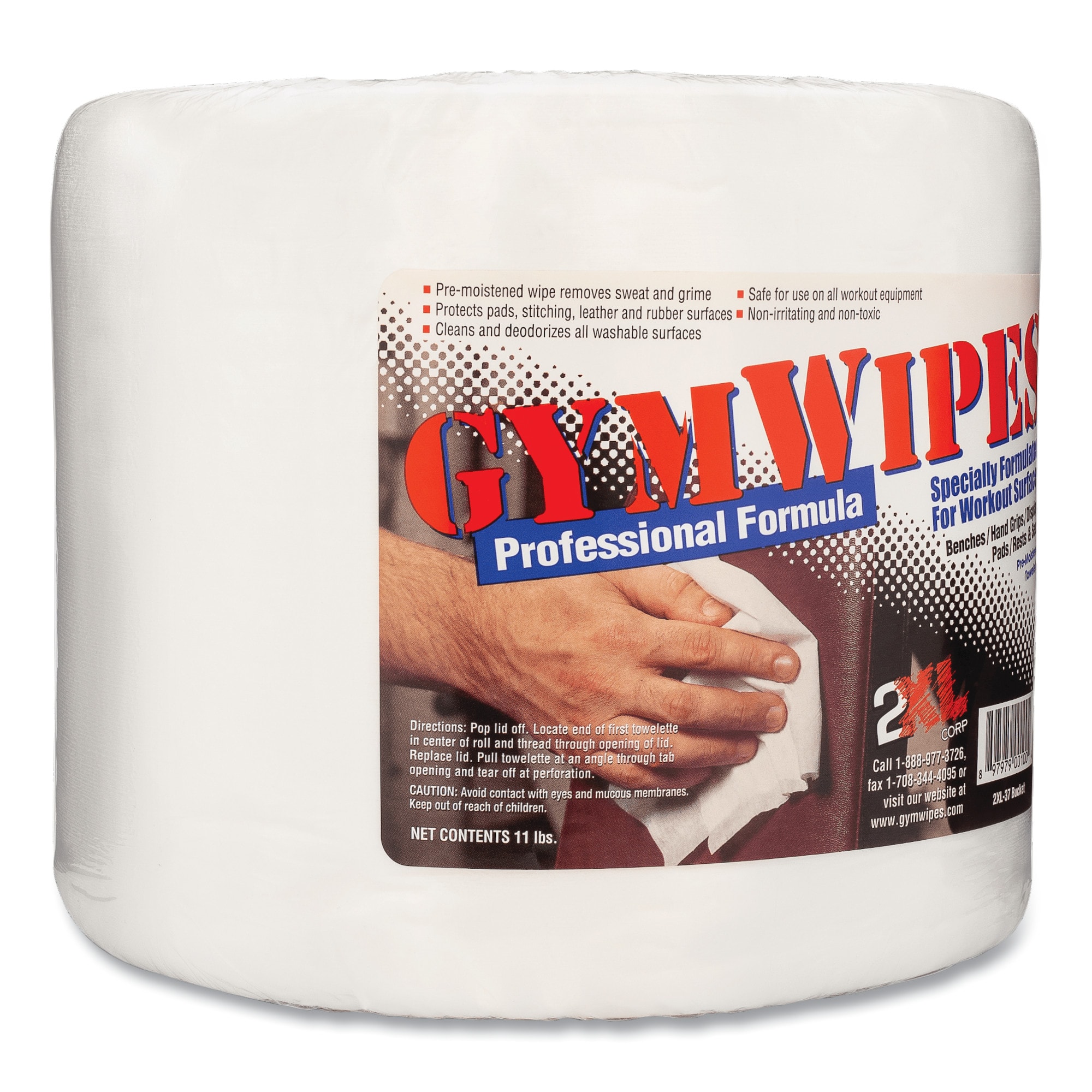This promotional image showcases a large, cylindrical package of pre-moistened gym wipes, prominently positioned in a stark, white void to draw all attention to the product itself. The wipes are packaged in a white container adorned with a detailed label. At the top of the label, bold red text reads "Gym Wipes," followed by a blue square highlighting the tagline "Professional Formula." The label features an image of a hand using a wipe to clean a brown or maroon surface.

Several bullet points emphasize the product's key features: it removes sweat and grime, protects pads, stitching, leather, and rubber surfaces, cleans and deodorizes all washable surfaces, and is safe for use on all workout equipment. Notably, the wipes are non-irritating and non-toxic, specially formulated for workout surfaces.

The bottom left of the label provides directions for use, explaining how to pop off the lid, locate the end of the first towelette, and thread it through the opening. It also lists cautions, including avoiding contact with eyes and mucous membranes and keeping the product out of reach of children. The net contents of the package are indicated as 11 pounds.

In the bottom right corner, a logo displays "2XL Corp" with "2" in white and "XL" in red, accompanied by contact information, including a phone number, fax number, and website. Additionally, a barcode with the number 9797900100 is situated on the label. This meticulously designed image serves to effectively communicate the benefits and usage instructions of the gym wipes, targeting potential buyers looking for professional cleaning solutions for workout equipment.